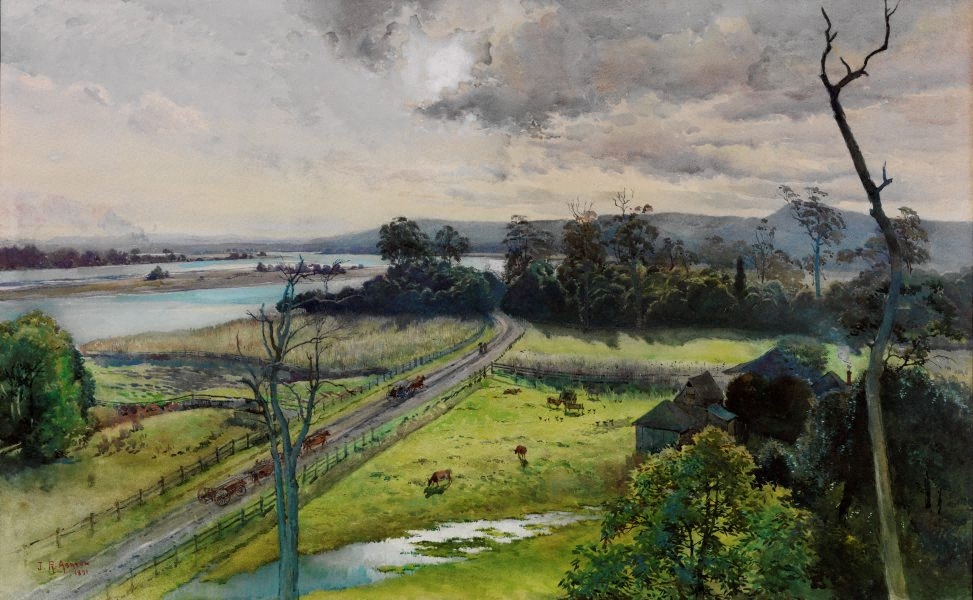This detailed painting of a farming landscape offers a panoramic view from an elevated vantage point, possibly from the top of a tall tree. In the background, a majestic range of mountains stands against a gray, overcast sky, while a winding road extends from the bottom left corner to the center, bordered by old-style wooden fencing. Along this road, a stagecoach and several horses, accompanied by two small figures, travel back and forth. To the left of the road lies a serene lake, while to the right, a lush grassy field hosts grazing cattle. Further right, near the corner of the image, a cluster of farm buildings is nestled amidst the greenery. A stream meanders through the scene, possibly hinting at recent flooding, and is flanked by tall grasses and wheat fields. Trees create a natural border in front of the mountains, and a small sandbar in a river or river confluence adds another layer of depth to this rich pastoral setting.